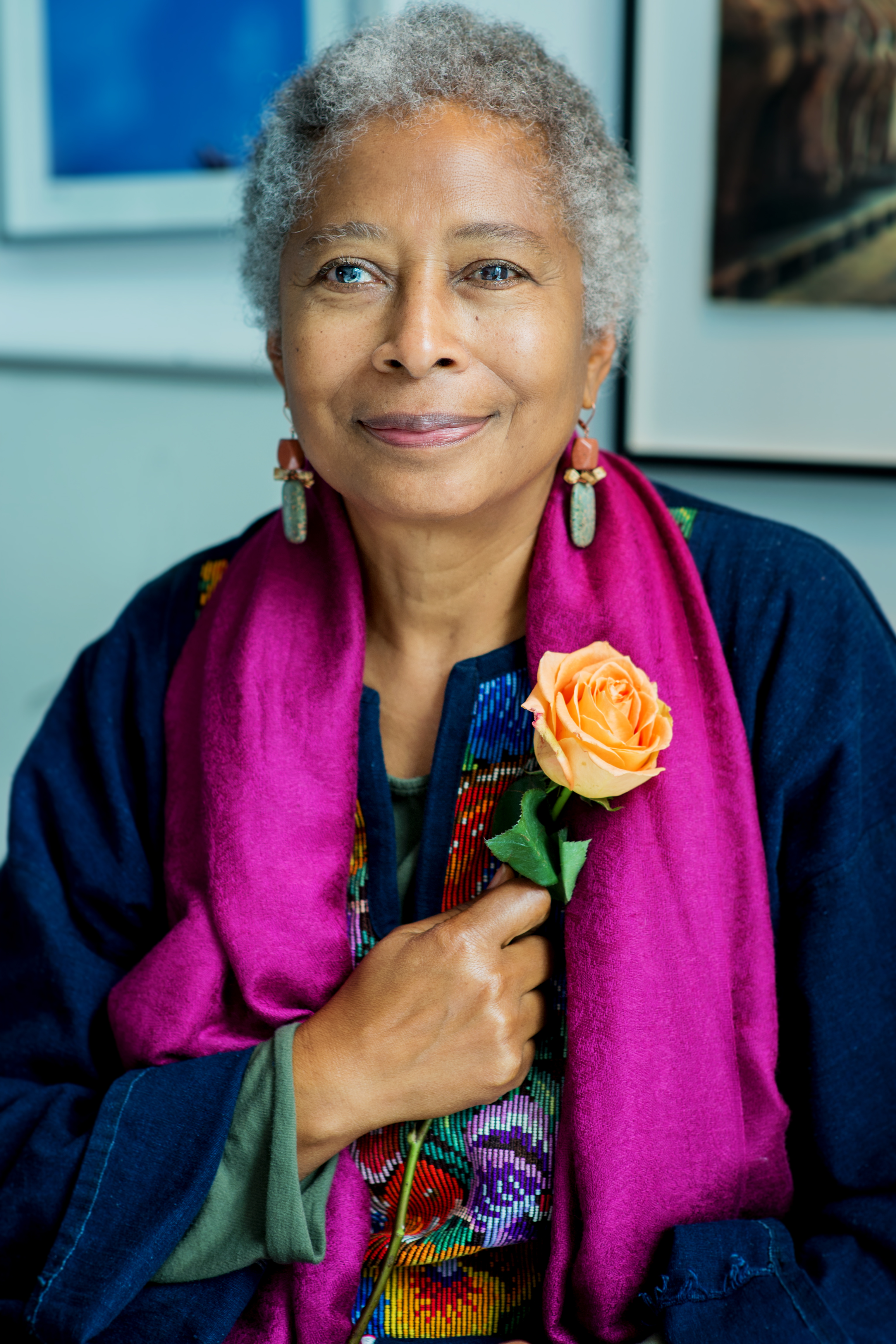This detailed photograph captures an elegant older African-American woman, likely in her 60s, posing with a soft smile that exudes warmth and grace. Her short, salt-and-pepper hair complements her smooth, brown skin, and she looks confidently into the camera with her striking, dark brown eyes—one of which intriguingly appears to have a segment that is blue, perhaps suggesting a genetic mutation or cataract.

She is adorned in a layered outfit that reflects rich cultural undertones. She wears a dark blue denim overshirt with a narrow V-neck, which features vibrant embroidery along the neckline, showcasing a bright array of flowers in blues, reds, purples, oranges, and greens. Underneath, a long-sleeve green shirt is visible, adding depth to her attire. Draped elegantly around her neck is a magenta scarf made of silk that adds a pop of color and aligns harmoniously with the hues of her embroidered top. She complements her look with a simple yet refined pair of stone and gold wire earrings.

Held gently in her right hand, close to her chest, is a delicate yellow rose whose subtle hue offers a beautiful contrast to her attire. The image's backdrop is subtle, featuring two out-of-focus framed photographs that add a personal touch without distracting from her presence. Despite her elegant and composed pose, there are some elements in the photo that appear slightly unnatural, potentially indicating that it might be AI-generated.

Overall, the image resembles a portrait typically used for promotional materials, such as an author photo accompanying an article or a brochure for an event where she might be speaking, encapsulating her poised and dignified demeanor.